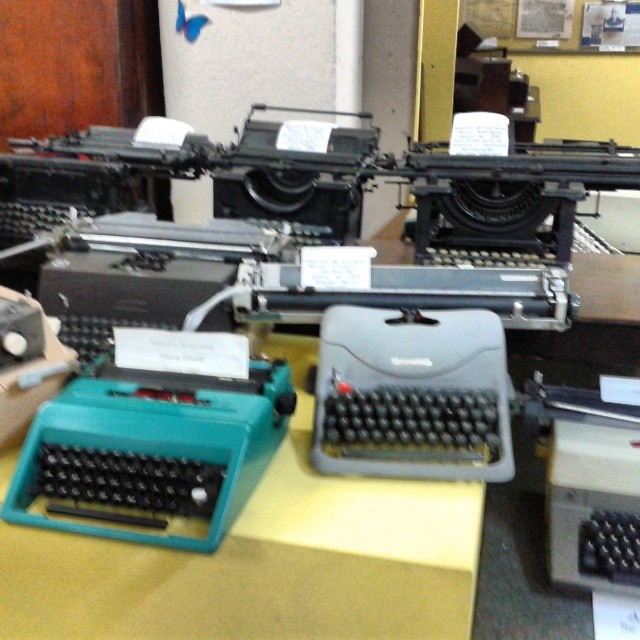The blurry square image captures a room filled with various typewriters arranged on desks. In the upper left corner, part of the yellow wall features a bulletin board covered with papers. Adjacent to this, a white wall with a decorative picture of a blue butterfly is visible. The room is set up with multiple rows of typewriters in different styles and colors: the back row showcases three black typewriters with papers inserted in them, the middle row has several gray typewriters, and the front row prominently displays a turquoise typewriter alongside a gray one, standing on a yellow counter, while the others rest on a brown desk. Additionally, there's a hint of a black machine that might be a copier and more posted papers in the upper right, adding to the sense of an old, cluttered workspace.